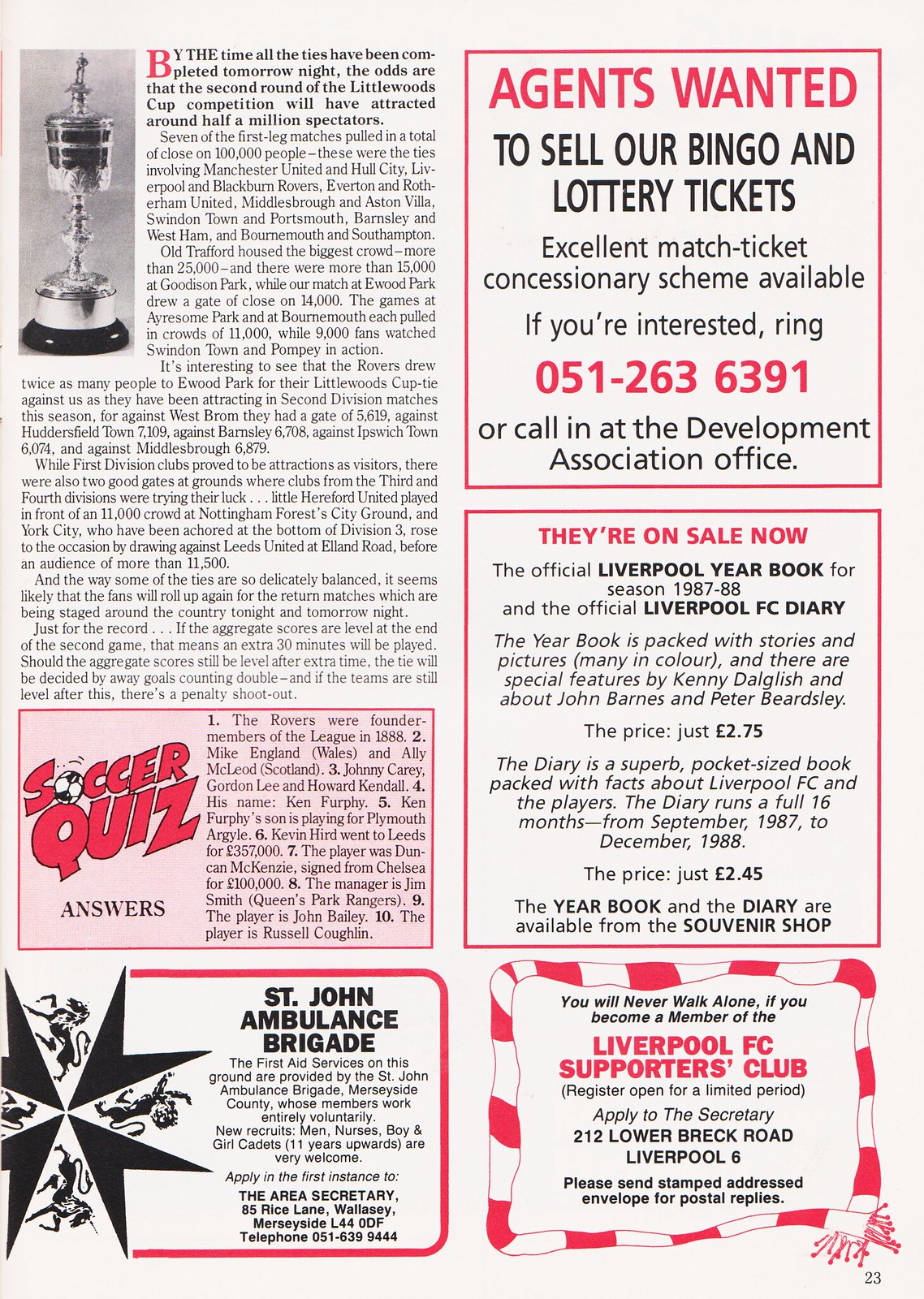This page from a vintage magazine, evocative of a 1950s style ad, is a detailed presentation of various elements connected to Liverpool FC and football events. On the left side, occupying approximately 80% of the upper two-thirds, is an article accompanied by a black and white image of a trophy, which looks like a chalice with a spire-like cover. The article discusses the widespread attention garnered by the second round of the Littlewoods Cup competition, which expects to attract around half a million spectators, highlighting matches involving notable teams such as Manchester United, Liverpool, and Everton.

Beneath the article on the left side, there is a pink-background text box featuring a "Soccer Quiz," where the letter "O" is stylized as a soccer ball. This section provides answers to trivia questions, such as noting that the Rovers were founding members of the league in 1888.

To the right side of the page, multiple advertisements are laid out. At the top right, a large text in red declares, "Agents Wanted to sell our bingo and lottery tickets." Below this, another advertisement announces, "They're on sale now," promoting the official Liverpool FC yearbook for the 1987-1988 season. Further down, an ad bordered by a red and white scarf—likely Liverpool FC colors rather than a Christmas motif—invites readers to join the Liverpool FC Supporters Club, with a note indicating that registration is open for a limited period.

On the bottom left of the page, a logo resembling a pointed star with interior lines marks the St. John Ambulance Brigade's advertisement, noting that first aid services on the grounds are provided by this organization. The entire layout is printed on a simple white background, giving the appearance of a traditional Liverpool FC handbill from a soccer match.